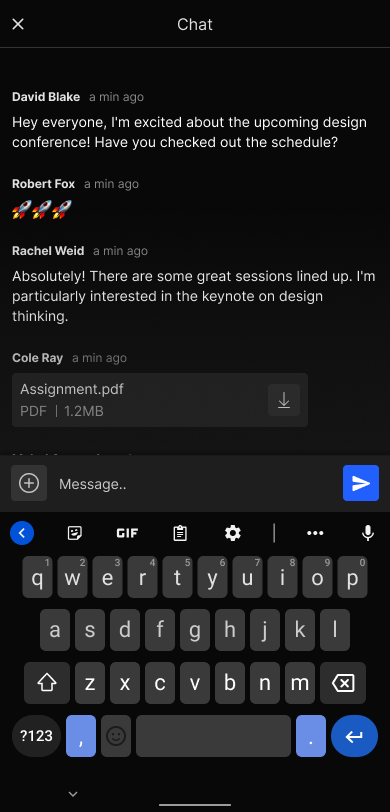This image is a vertical screenshot from a mobile phone, showcasing a real-time chat interface. At the top center, it displays the title "Chat." Below this, several participants' messages are visible, each timestamped from a minute ago. The chat begins with David Blake who says, "Hey everyone. I'm excited about the upcoming design conference. Have you checked out the schedule?" Robert Fox responds with three diagonally arranged rocket emojis in blue, red, and yellow. Rachel Weed follows with, "Absolutely. There are some great sessions lined up. I'm particularly interested in the keynote on design thinking." The next message is from Cole Ray and includes an attachment labeled "assignment PDF," which is downloadable through a designated box. 

Approximately two-thirds down the screen, there's a message input bar. This bar is gray, with a circle and plus sign on the left for adding attachments, a placeholder text that reads "Message..." in the center, and a blue square on the right featuring a right-facing arrow for sending the message. Below this, the on-screen keyboard is visible, ready for typing.